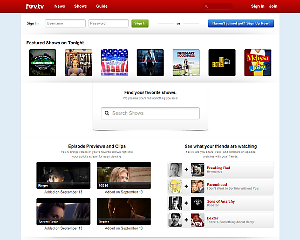The image depicts a blurred screenshot of a TV platform website, characterized by a red title bar with the phrase "something TV" located in the upper left-hand corner. The site features a navigation menu consisting of three buttons on the left and two additional options on the right, one of which appears to be a sign-in button. 

Below the navigation menu, there are two rectangular boxes followed by a green button, another input box, and a blue button. Further down, the layout includes a row of seven small boxes, each containing an image. A white rectangular search bar is situated beneath this row of icons.

At the bottom of the screenshot, there are more images organized into rows. On the left-hand side, a series of images are displayed, while on the right-hand side, there are two rows, each containing a single image with a plus sign next to it.